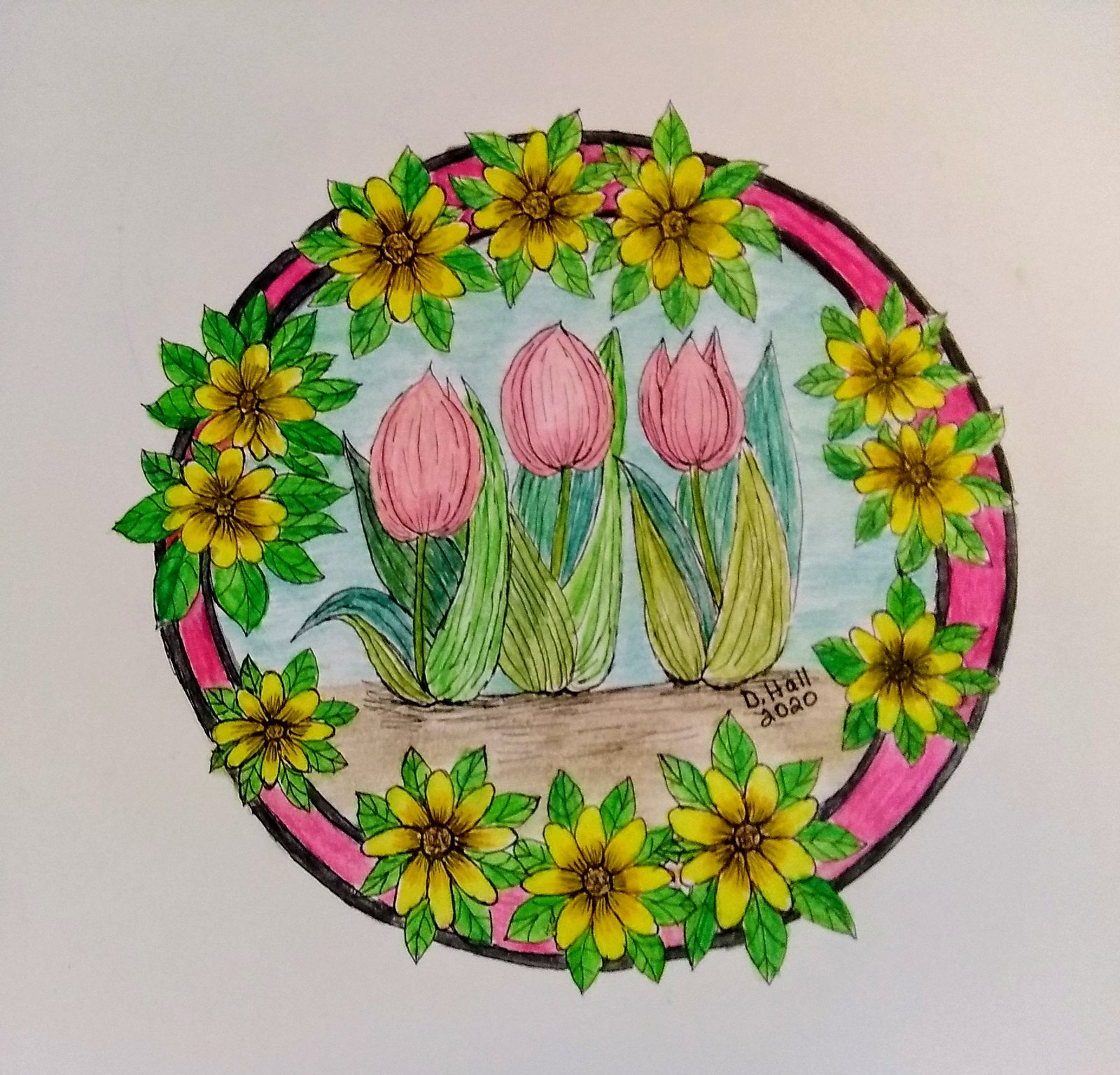A captivating artwork by D. Hall, created in 2020, showcases a beautiful illustration of three fully bloomed pink tulips. These elegant flowers are encircled by small, yellow daisy-like blossoms, set against lush green leaves. The entire scene is enclosed within a delicate pink frame that evokes the appearance of stained glass. The background features a soft, pastel pink hue, contributing to the overall serene and charming aesthetic. This exquisite piece, with its intricate details and harmonious colors, would make a delightful addition to any wall, offering a sense of timeless beauty and refined artistry.